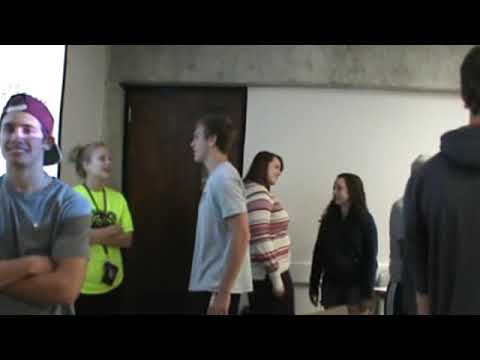The photograph features a lively group of about seven college-age students socializing in what appears to be a classroom setting with gray cement walls, a large whiteboard, and a brown door on the left. The scene exudes a casual, almost party-like atmosphere, with students engaged in conversation. 

On the far left, a young man stands with his arms crossed, wearing a backward red (or possibly purple) baseball cap and a t-shirt, smiling. Just behind him, a young woman with blonde hair pulled back into a bun, dressed in a yellow shirt, is engaged in a conversation with a tall young man in a gray t-shirt and shorts. They are all casually dressed, exchanged between each other in lighthearted discussions.

To the right of these students are two young women immersed in their conversation. The woman on the left wears a red and white striped shirt and black pants, with long black hair, while her companion is dressed entirely in black with similar long brown hair. Further to the right, another young man stands with his back to the camera, hinting at the informal and dynamic interaction among the group. The photograph captures a moment of cheerful interaction among the students, highlighting their youth and camaraderie.